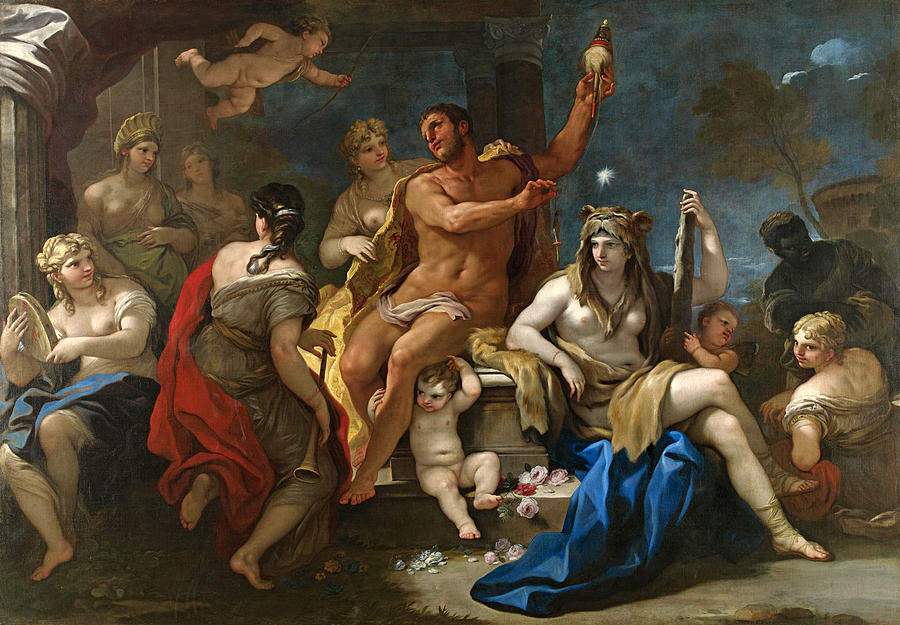The painting depicts an ancient scene, possibly of Greek or Roman inspiration, centered around a male figure who appears to be of significant importance, potentially a king. This man, partially draped in a cloth and possibly a cape, sits on a platform or step with his left leg extended over a naked child who clings to it. He has short hair, a beard, and holds an object, perhaps a bird, up towards the sky. At his feet rests another baby, and to his left, a naked cherubic figure floats, reminiscent of a baby angel. Surrounding the central figure are numerous women, many of whom are partially clothed in draped fabrics or togas that leave their breasts exposed. One standout is a blonde woman adorned with earrings and a covering over her shoulders, gazing at the central man. In the background, several other topless women look towards him, some with smiles. The backdrop includes what appears to be a pillar and possibly a rocky or coffin-like structure. Off to one side, an individual, potentially an African-American man or someone shrouded in shadows, adds a subtle contrast, though they do not appear to be the focus of the scene. The overall composition emphasizes the central male figure and the surrounding women and children, creating a dynamic and detailed tableau evocative of classical antiquity.